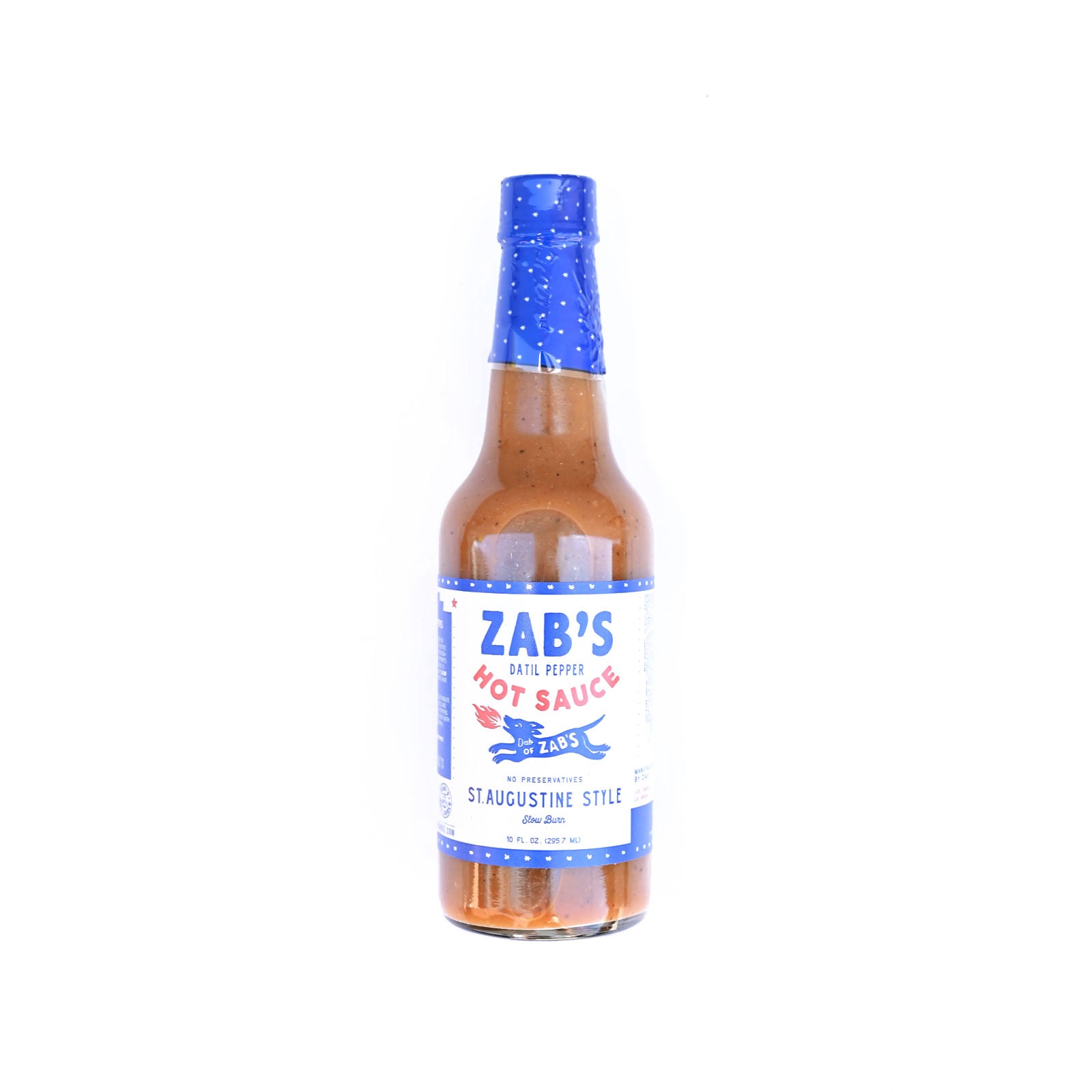The image showcases a bottle of Zab's Datil Pepper Hot Sauce, prominently displayed against a white background. The hot sauce is contained in a clear glass bottle that resembles the size of a beer bottle and features a slender neck. The top of the bottle is wrapped in a blue foil with tiny gold polka dots and is trimmed with gold at the bottom, extending down the neck. The sauce within is a rich, medium brownish-red color, speckled with visible pieces of pepper. The label, which is similarly blue with gold polka dots, displays the brand name "Zab's" in bold blue letters, with "Datil Pepper" written underneath. The label also includes red text stating "hot sauce" and highlights the product's key features, such as "No Preservatives" and "St. Augustine Style, Slow Burn." The logo features an illustration of a dog spewing fire and the phrase "dash of Zab's." Across the top of the label, the bottle’s cap appears to be unscrewed, revealing more of the hot sauce inside.